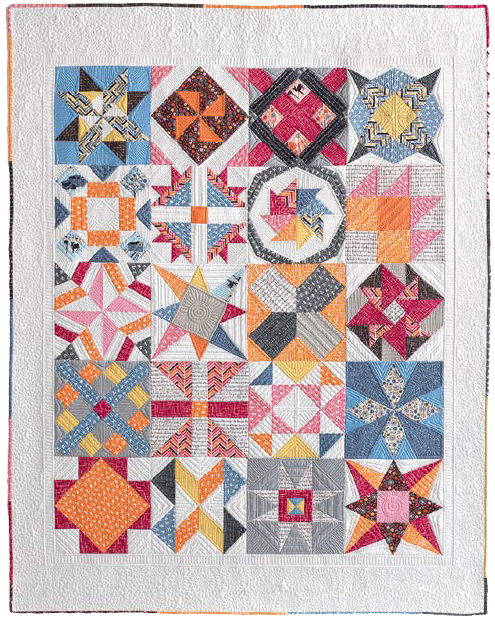This is a top-down photo of a handmade quilt with a grid pattern consisting of four columns and five rows, featuring a total of 20 unique squares. Each square showcases distinct patterns predominantly in burst and windmill shapes, incorporating colors such as blue, yellow, orange, pink, red, black, and gray. The quilt sits atop a white, lacy, doily-textured fabric, surrounded by a thin border made from scrap pieces matching the internal quilt colors, which include black, red, yellow, and blue. The quilt's design combines various geometric shapes like triangles, diamonds, and squares, with a significant amount of intricate texture and color variation, making each patch distinct and vibrant.